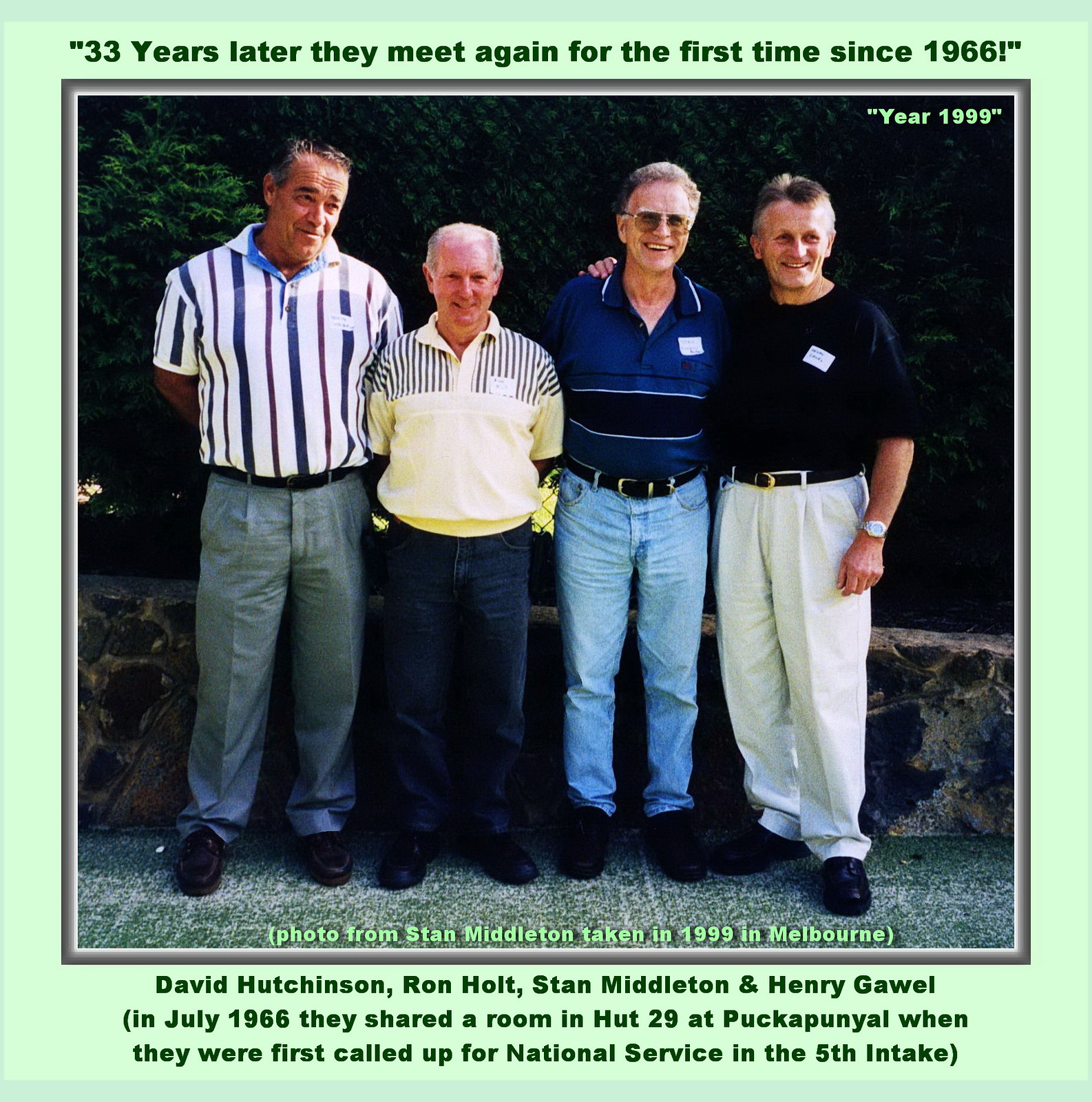The image features a cherished reunion of four elderly men—David Hutchinson, Ron Holt, Stan Middleton, and Harry Cowell—standing closely together, smiling warmly. These men, who first met in 1966 when they shared a room in Hut 29 during their national service in the 5th Intake in Australia, are gathered again for the first time in 33 years. The photograph, marked with the year "1999," captures this heartfelt moment.

From left to right:
- David Hutchinson, the tallest, is dressed in a white shirt with blue and purple stripes and beige pants.
- Next to him stands Ron Holt, a shorter gentleman with white hair, wearing a white shirt and blue slacks.
- Stan Middleton, an older man sporting sunglasses, wears a blue polo shirt with deep navy stripes and blue jeans.
- Lastly, Harry Cowell is clad in a black t-shirt and white pants.

Behind them, a stone sidewalk and wall are visible, with a fence and dense, dark green pine trees providing a lush backdrop. The caption at the top of the image poignantly reads, "33 years later they meet again for the first time since 1966," highlighting the enduring bond of these four friends.